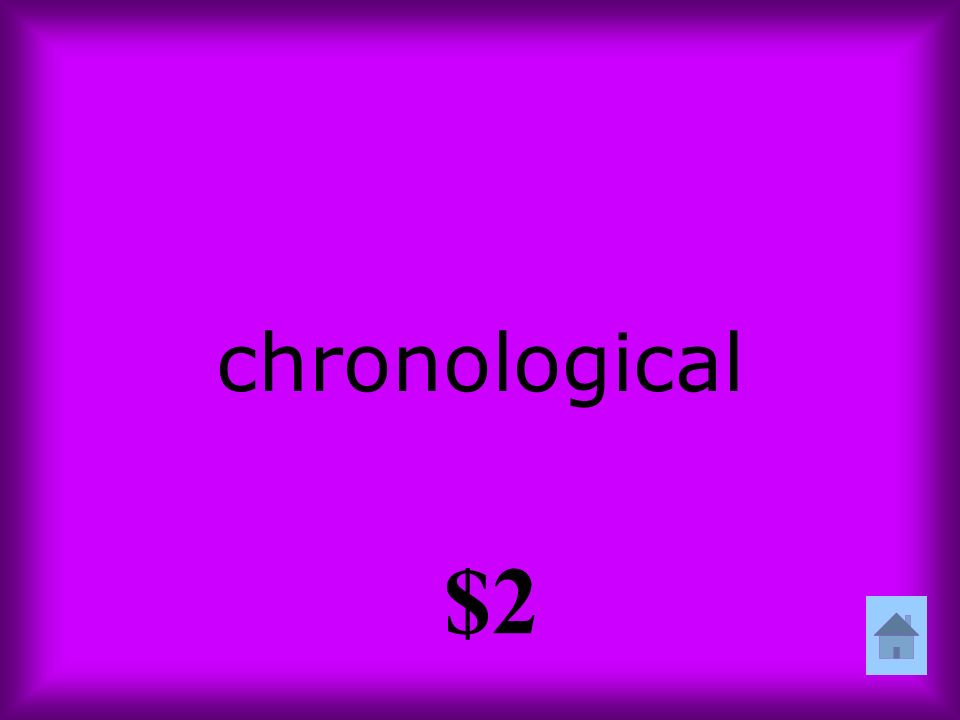The image features a square purple background with an embossed effect, transitioning from a darker purple at the edges to a lighter purple towards the center. Prominently displayed in small, all-black lowercase letters in the center is the word "chronological" (spelled C-H-R-O-N-O-L-O-G-I-C-A-L). At the very bottom center, a black dollar sign followed by the number 2 indicates a price of $2. In the bottom right corner, there is a small, light gray square containing a simple 2D silhouette of a house. The house has a square base, a triangle-shaped roof in dark gray, a rectangle door, and a square chimney, all outlined in slightly darker shades. The design suggests a simplified, possibly game-like graphic.